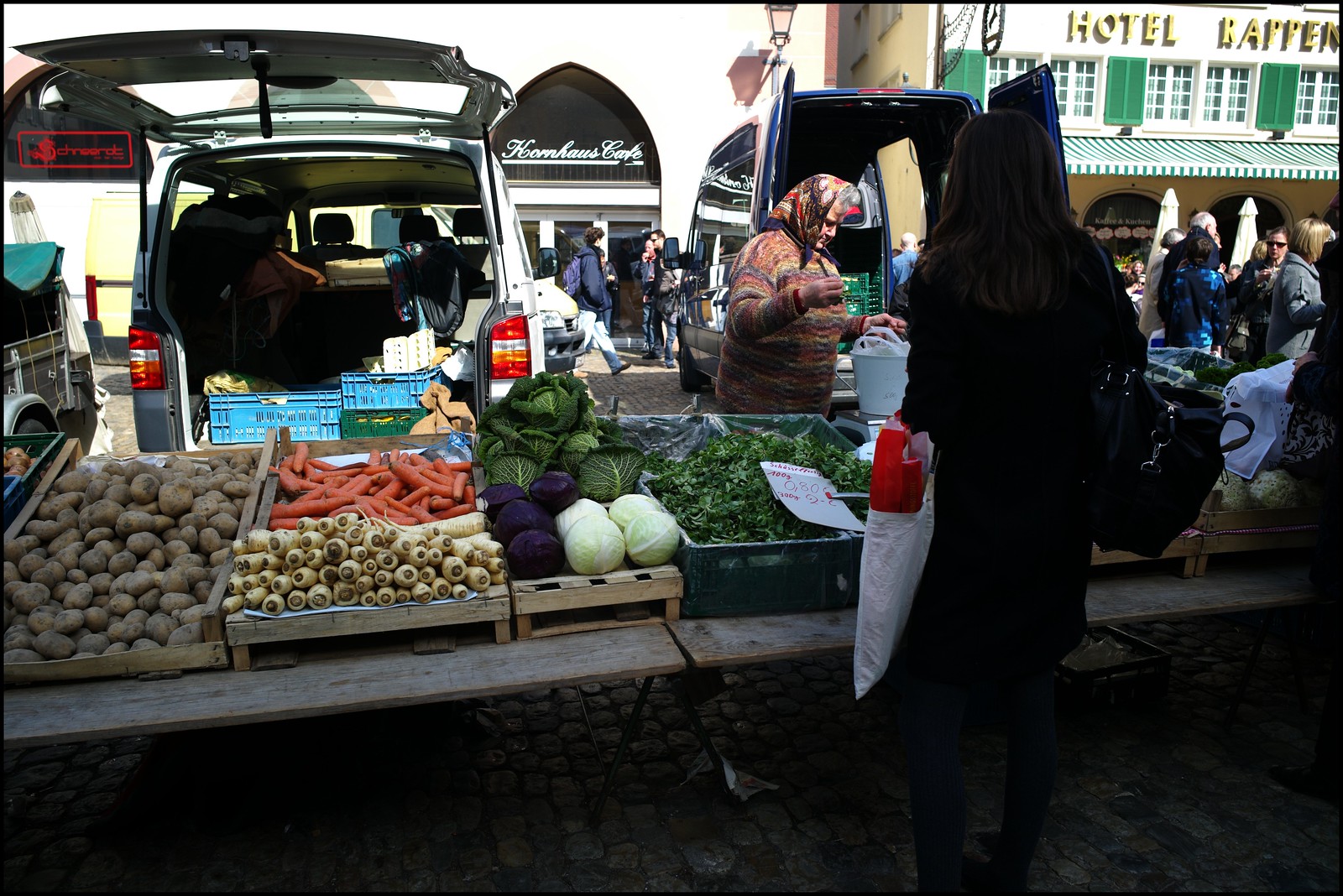The image depicts a vibrant outdoor street sale brimming with activity. In the foreground, a shopper dressed in dark clothing stands facing a makeshift vegetable display, intently examining an assortment of produce including potatoes, carrots, parsnips, green cabbage, purple cabbage, light green cabbage, and squash. She holds a white bag with something red protruding from it in her left hand and a black bag in her right hand. The vegetables are neatly arranged on wooden tables supported by pallets and stacks of logs, creating a rustic market setup. 

To her left, an older woman in a scarf appears to be either shopping or working. Behind them, more people bustle along the busy city street, enhancing the dynamic atmosphere. The background reveals the facade of a building with the Hotel Rackenne, marked by its distinct green shutters and an overhanging shade, and the Kuhn House Cafe further down the street. Adding to the scene’s liveliness, two vans with open back doors are parked nearby, with crates of produce being unloaded into the market. Several closed umbrellas suggest a temporary setup, typically seen in such bustling farmer's markets. The bright, sunny weather further illuminates the entire scene, casting shadows and highlighting the vibrant colors of the fresh produce on display.